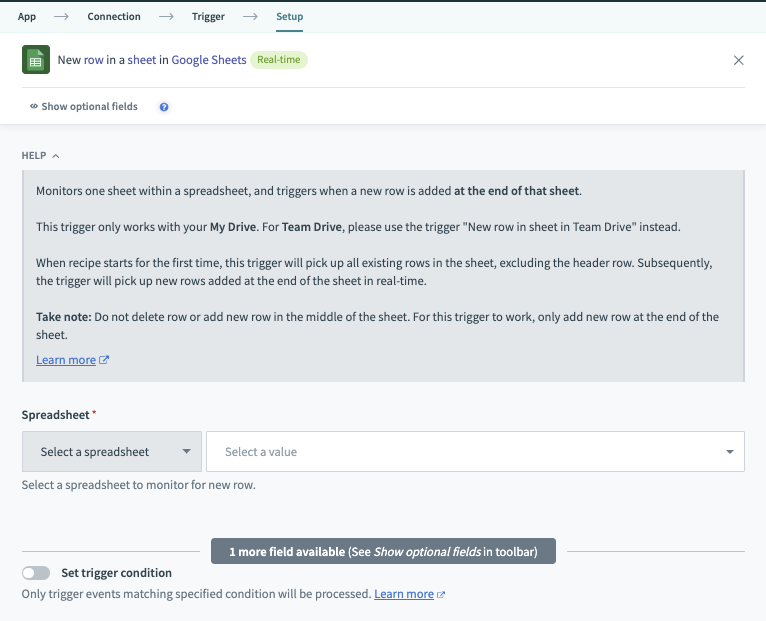The image displays a help section within the Google Sheets interface, specifically focused on setting up a trigger for monitoring a sheet. The top portion of the screen reads "Monitor: New row in a sheet in Google Sheets," indicating that the feature tracks and triggers actions when a new row is added to the end of the specified sheet. 

The help text elaborates that this trigger only functions with Google Drive. A section labeled "Set Trigger Condition" suggests that only events matching specific conditions will be processed, and notes that this feature can be toggled on or off—the current status shows it is off.

Below, there is a dropdown menu labeled "Select a Spreadsheet," which is currently empty. The top menu navigational path shows "App > Connection > Trigger > Setup," hinting at the steps needed to configure this trigger. Additionally, an option mentions, "One more field available: show optional field in toolbar," suggesting additional customization for more advanced users. The overall visual implies that this help section is aimed at users seeking to understand and utilize advanced trigger functionalities within Google Sheets.